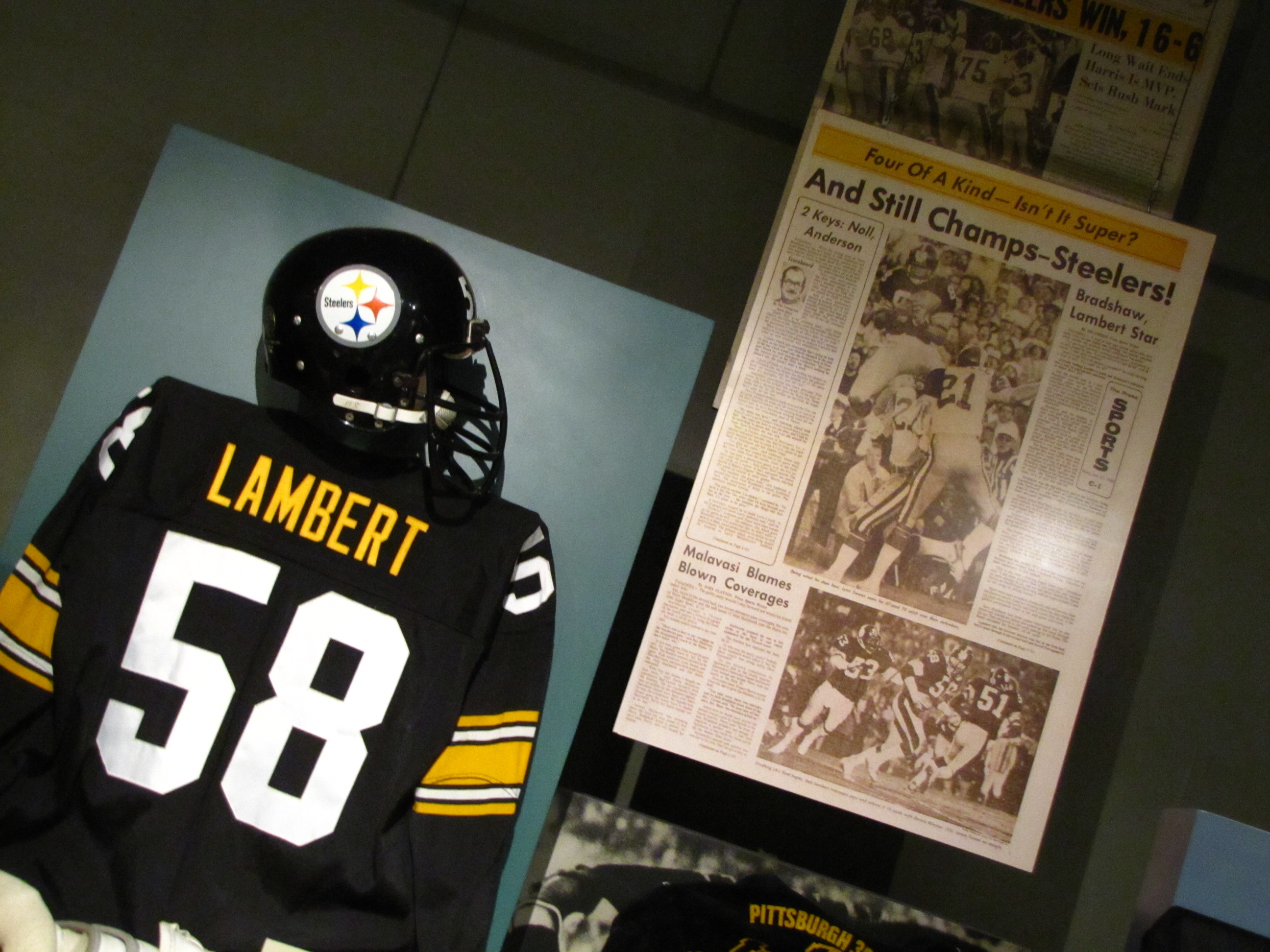The image depicts the back of a black football uniform prominently displaying the white number 58 and the yellow name "Lambert" above it. Yellow and white stripes adorn the sleeves, and a dark helmet, featuring a white circle with "Steelers" in black text and an inverted diamond shape in yellow, orange, and blue, is positioned above the jersey. The scene is set against a light blue background, with a newspaper article nearby. The headline reads, "And Still Champs - The Steelers," and features a horizontal, rectangular photo of a football game, along with black-and-white pictures and written articles. The composition suggests a display or section of a board dedicated to football memorabilia.